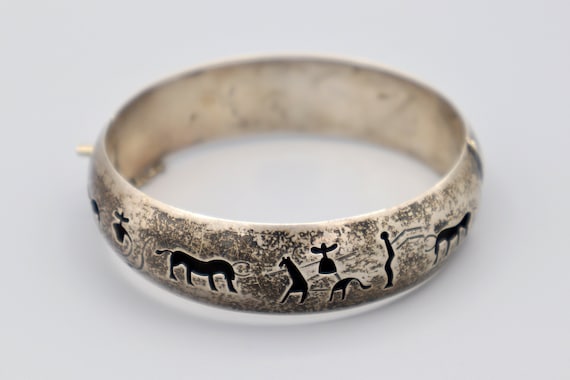This image showcases a large, aged ring with a scuffed, rusty appearance, set against a light beige or very light gray background. The ring appears to be silver, although some areas reflect a gold-like hue, indicating possible discoloration or dirt accumulation over time. The exterior is adorned with silhouettes of various figures, including animals and humans, all in a dark color palette ranging from deep black to dark brown. On the left side of the ring, there is a black lion-like figure followed by what resembles a giraffe with a long neck but not significantly taller than the lion. To the right of these animals, there is a figure that appears to be a person wearing a wide-brimmed hat, followed by a stick figure, and another animal. The interior of the ring remains plain, without any engravings or additional designs. The combination of these worn, dark silhouettes and the ring's tarnished surface suggests a piece that has aged and perhaps been well-worn over time.